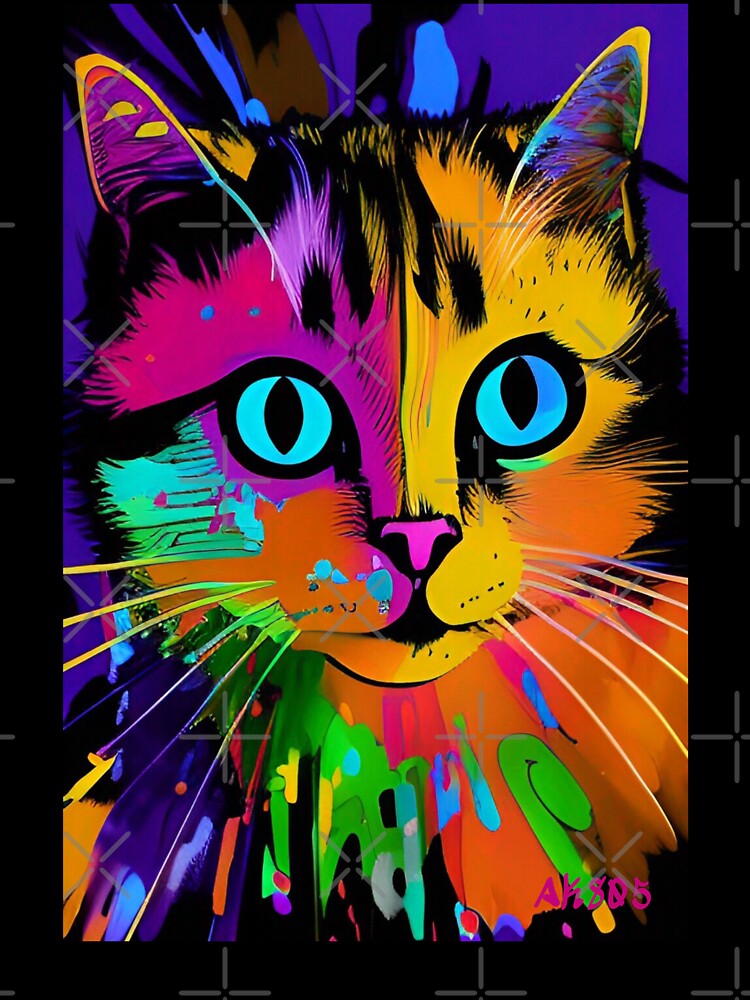This tall, rectangular digital artwork, framed with thick black borders on the left, right, and bottom edges, captivatingly showcases a vibrant, rainbow-colored cat against a purple-black backdrop. The focus is on the cat’s face, which prominently fills the width of the image, while the body extends and gets cut off on the right side. The left side of the cat's face features rich pink and purple hues accented with black shadows, while the right side bursts with bright yellow and orange. Delicate, yellow-bordered rainbow ears, a bright pink nose, and luminescent neon blue eyes add to the cat's whimsical charm.

A detailed, layered texture of alternating transparent gray plus and multiplication signs overlays the scene, adding depth and complexity. The cat’s whiskers are light yellow, while splattered green paint adorns the bottom of the image, merging with splashes of purple and blue. A subtle watermark of repeated gray lines is noticeable throughout the artwork, and the bottom right corner bears a distinctive pink signature, "AK-805," which could hint at the artist's identifier, enhancing the piece’s authenticity. The creativity and colorful vibrancy make the cat appear animated and cartoonish, yet absolutely captivating.